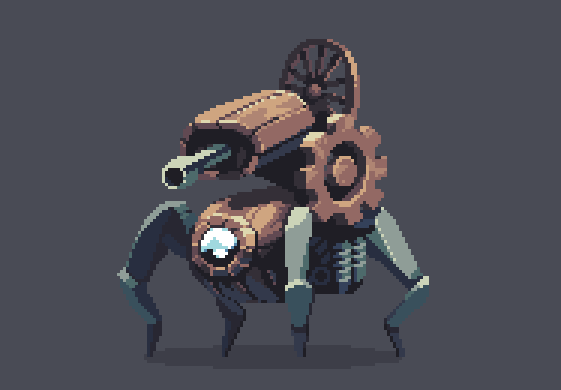The image depicts intricate pixel art of a small, mechanized robot with a distinctive cybernetic, steampunk appearance. The robot features a prominent lens in its center, resembling an illuminated white camera eye, mounted on a reddish-orange body with a bluish backside. It stands on four spider-like legs that are colored in varying shades of gray, blue, and dark green. Attached to the robot’s back is a large cogwheel with spokes, alongside a second wheel that resembles a wooden wagon wheel, connected by a lever mechanism. Atop the machine, a futuristic turret gun is mounted, though it’s unclear whether this is an actual gun, laser, or flamethrower. The artwork is set against a dark gray background, with a small shadow cast beneath the robot, adding to the depth and detail of the piece.